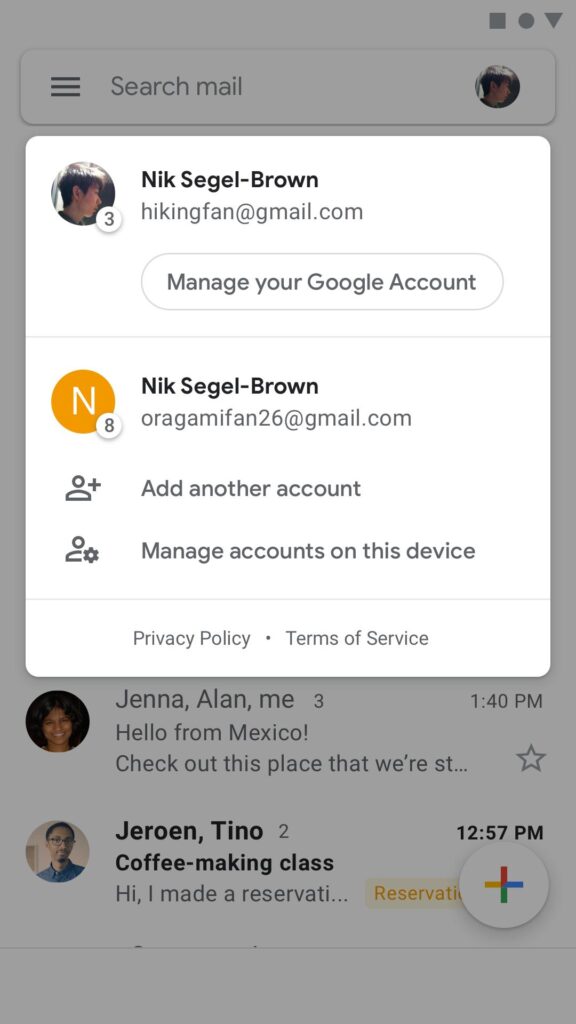In this image, we see a screenshot overlaid by a pop-up box. The box is prompting the user to manage their Google account, displaying options such as "Nick Siegel, Typhon, Brown," along with the associated email addresses: hikingfan@gmail.com, nicksiegelsmichbrown, and gammafan26@gmail.com. The user can also add another account or manage accounts on the device. 

In the background, there is a list of emails. One visible email is from Jenna to Alan, marked "me," with the timestamp 3:1.40 PM in Hilo, New Mexico, discussing the place they are staying at. Additionally, there's a notification about an upcoming coffee-making class. The interface shows typical footer options like "Privacy" and "Terms of Service."